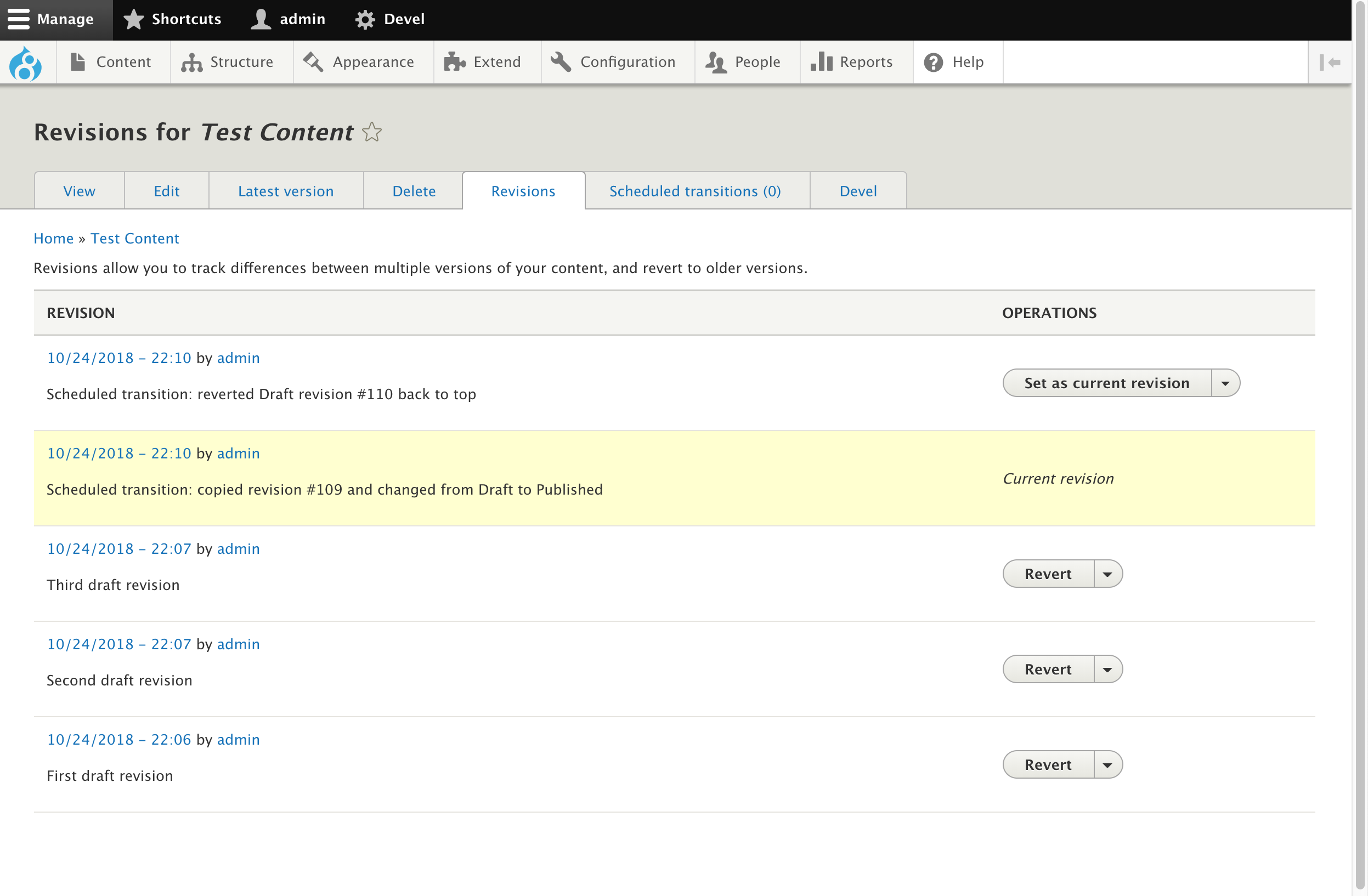The image depicts a website interface. At the top, it features a navigation bar with a hamburger menu icon, followed by options for Manage, Shortcuts, Administration, and a settings gear icon labeled Development. Below this bar, there is a logo that appears to be a blue teardrop with a symbol that could be interpreted as a slanted '8', a 'G', or an ampersand.

Beneath the logo, a secondary menu includes Content, Structure, Appearance, Extend, Configuration, People, Reports, and Help. Directly under this menu, a section titled "Revisions for Test Content" offers various actions such as View, Edit, Latest Versions, Delete, Revisions (currently selected), Schedule, Transitions, and Development.

The content area explains that "Revisions allow you to track differences between multiple versions of your content and revert to older versions." Below this explanation, the layout splits into two columns: Revision and Operations. The first entry is dated October 24th, 2018, at 10:10 by Administration. It includes options to Schedule, Transition, Revert to Draft Revision #110, and is marked as "Set as current revision." The current highlighted revision is also from the same timestamp, labeled "Current Revision." Other entries list additional draft revisions (third, second, and first drafts), although they appear similar in content.